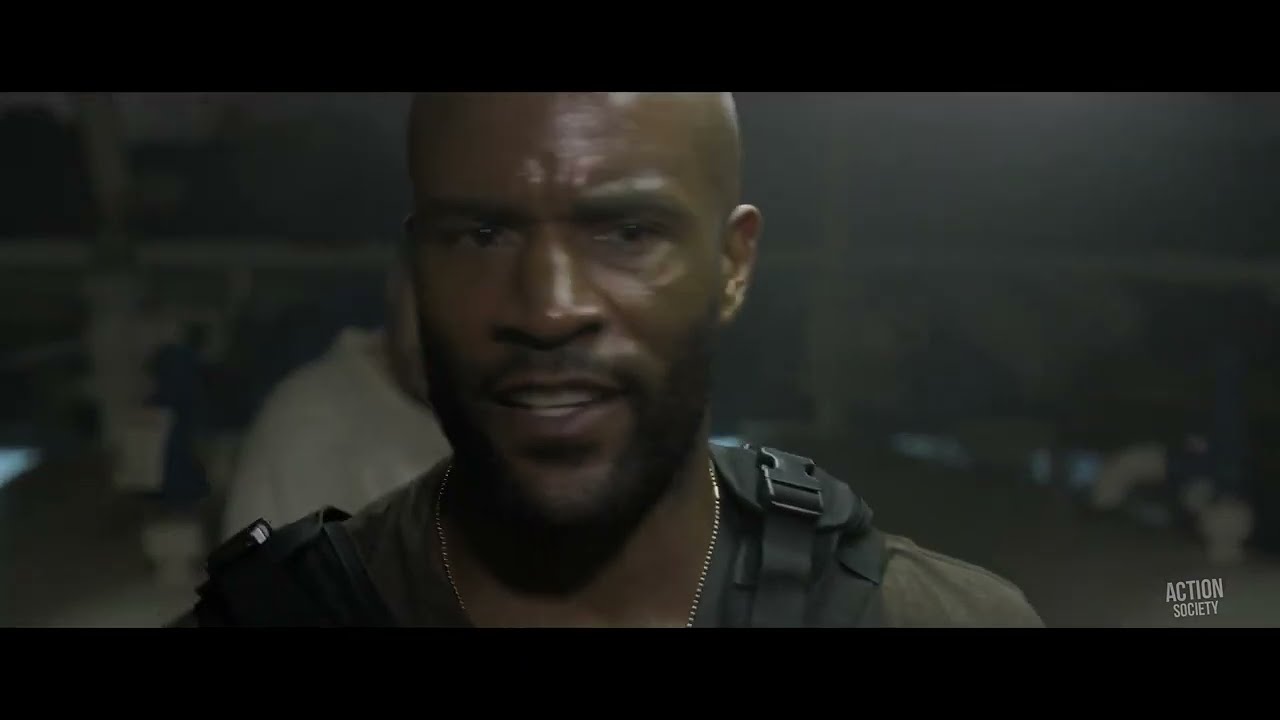The image depicts a serious-looking man of African descent, centered in the frame, with a bald head and a slightly open mouth revealing both his upper and lower teeth. His dark skin glistens with sweat, highlighting his prominent black mustache and beard. He is dressed in a greyish-brown t-shirt and has black straps across both shoulders, likely from a backpack, along with a silver necklace made of tiny beads or a dog tag-like chain. The scene has a cinematic quality, possibly a screenshot from a movie or video, with the man's upper shoulders to the top of his forehead visible, framed by black horizontal strips above and below the image. In the blurred background, hinting at a dim and messy environment, stands another person wearing a white t-shirt. The lower right-hand corner of the image bears a white watermark reading "Action Society."